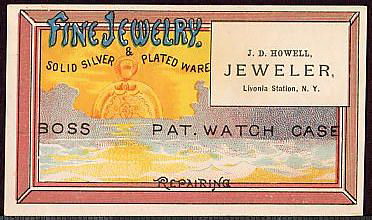This image depicts a vintage business card or advertisement with a visually rich, multi-layered border. The outermost border is black, followed by a white border, and then a red border. The card prominently features text and imagery denoting the services of J.D. Howell, Jeweler, located at Livonia Station, New York. 

The upper left corner is marked by the phrase "Fine Jewelry, Solid Silver, and Plated Ware" in blue text. The upper right corner contains a squared area with the jeweler's name, location, and presumably their logo. 

The central section of the card showcases the text "Boss Pat Watch Case," with the word "Repairing" located at the bottom center. The centerpiece of the card is a striking, creative image resembling a pocket watch emerging like a rising sun from a body of water, accentuated with shades of gold and an array of colors including black, tan, brown, blue, yellow, orange, and light blue. The overall design suggests an old-fashioned advertisement, rich in detail and evocative of a classic artisanal style.